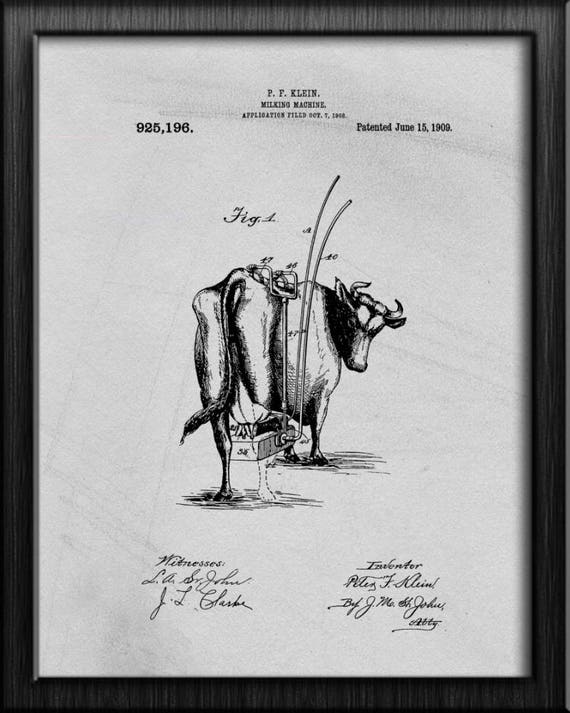This is a detailed black and white technical drawing of a cow, showcasing an early milking machine invention. At the top center of the image, the text "P.F. Kline" is prominently displayed. Beneath this, the label "Milking Machine" appears, followed by the application filing date of either October 7, 1908, or 1906. To the left side of the image, the patent number "925,196" is listed. On the right side, the patent approval date "June 15, 1909" is noted. Above the cow, the label "Figure 1" identifies the illustration.

The cow is depicted from a rear view, allowing a clear perspective of the udder. The cow’s head is turned to look towards the viewer. Attached to the udder is a metal box-like milking device, from which several hoses or pipes extend. Two hoses rise above the cow, and another extends to a separate metal fixture located on the cow's back.

Beneath the cow, on the left side, the word "Witnesses" is followed by two signatures: "L.A. Senior John" and "J.L. Clark." On the right side, the term "Inventor" is followed by the name "Peter F. Kline." Underneath Kline's name appears another signature or annotation, "by J.M." with the rest being partially illegible.